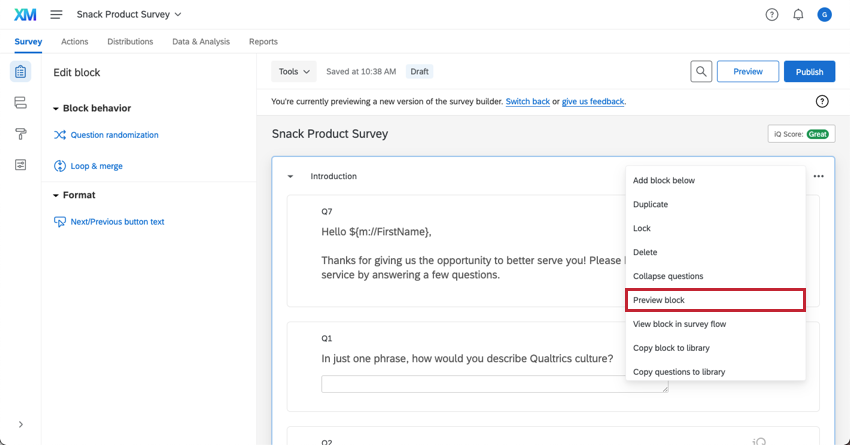Here is the refined and detailed caption for the image:

---

The screenshot captures the user interface of a website or application primarily designed with a white background, featuring text in black, gray, and blue. In the upper left corner, there is a blue section with black letters that read "XM." Adjacent to this is a black three-line menu icon, with the label "Snack Product Survey" placed beside a downward-pointing arrow, indicating the presence of a drop-down menu.

On the top-right side of the interface, there are three icons: a question mark encased within a circle, a notification bell, and a blue circle containing either the letter "G" or "Q." Below these icons is the primary navigation menu comprising the options: "Survey," "Actions," "Distributions," "Data & Analysis," and "Reports." The "Survey" tab is highlighted in blue and underlined, signifying it is the currently selected menu item, while the rest are displayed in black.

Following the selection of the "Survey" tab, an additional sub-menu appears below it, comprising four icons. To the right, there are several fields labeled: "Edit Block," "Block Behavior," "Question Randomization," "Loop & Merge," "Format," and "Next/Previous Button Text."

Dominating the main body of the screenshot is the header "Snack Product Survey," followed by a draft introduction script. This draft includes section headings aligned with the content, marked as "Q7," "Q1," and "Q2."

---